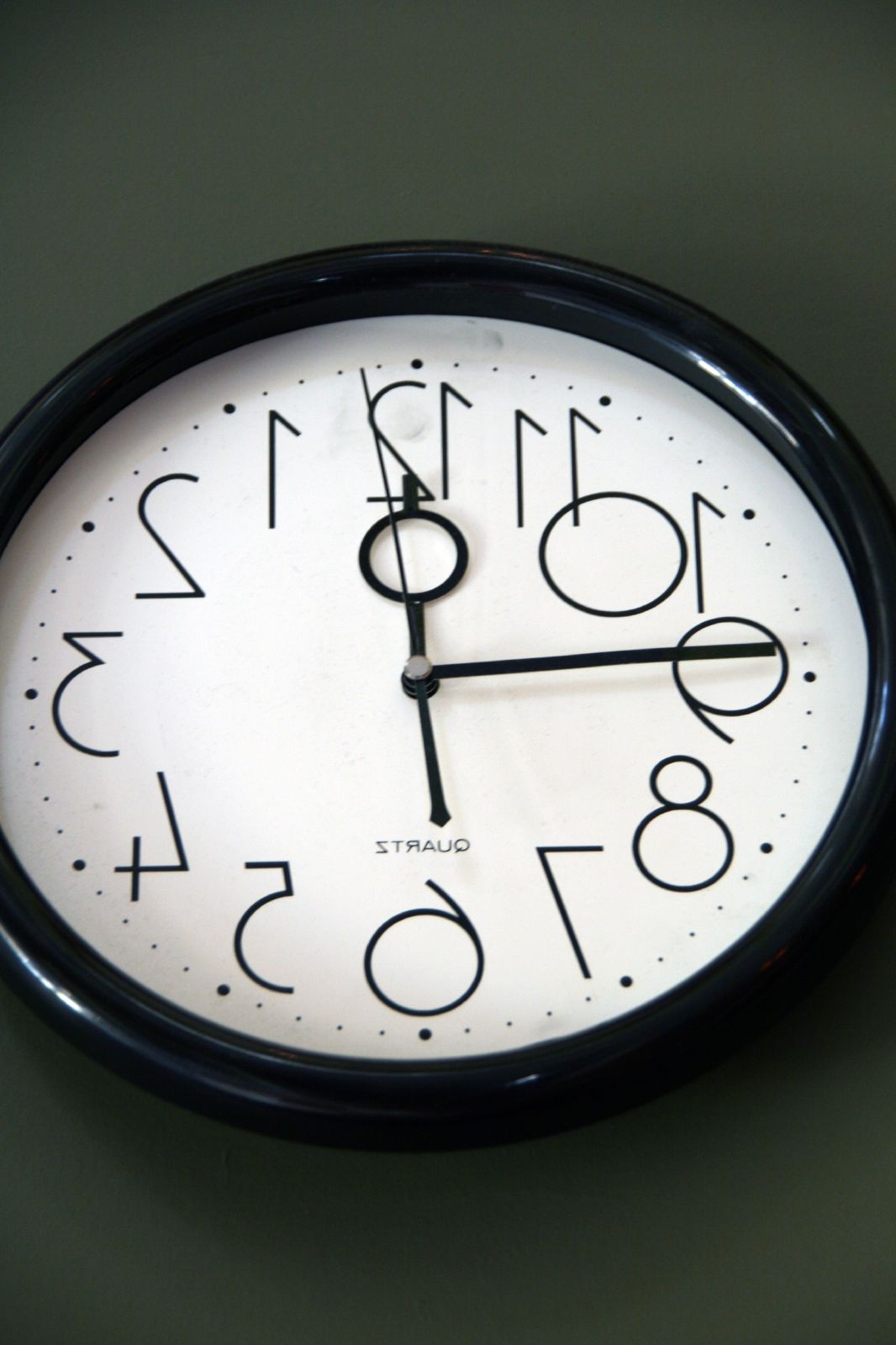The image features a circular clock hanging on a dark green wall, which appears smooth and deep olive in color. The clock's black, almost plastic-looking border is slightly cut off on the left and right sides, yet its circular shape remains identifiable. The clock face is white with large Arabic numerals from 1 to 12. It is mirrored, resembling as if you were looking at it in a reflection, making the numbers appear backwards. Small black circles mark the hours while even smaller ones indicate the minutes between. The hour hand is distinctive, with a straight line ending in a circle, then continuing straight to its end. The minute hand is a simple straight black line, and there is also a black second hand. The clock reads approximately 12:45, and the word "quartz" is visible at the lower part of the clock face, albeit in reverse.